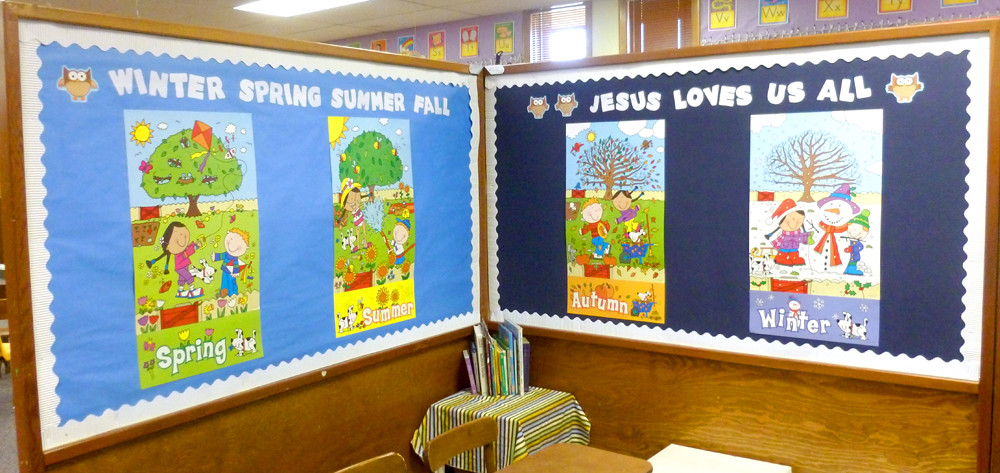The image captures a wide, horizontal view of the interior of a school building. At the top, there's a beige drop ceiling, approximately 12 feet tall, adorned with fluorescent lighting. The back right side of the image shows part of a wall, distinguished by purple paper trimming and several yellow signs featuring black text, spelling out "S-T-U" and "V-W-X-Y" with both uppercase and lowercase letters. A window in the center of the back wall looks out to a sunny day, as evidenced by the light streaming in.

In the central area, there's a small display cubicle made with a light brown wood frame. To the left of this cubicle, a light blue sign measuring about four feet tall and eight feet wide reads "Winter, Spring, Summer, Fall" in white text, bordered with white trim. Adjacent to it, a dark blue sign with similar dimensions and trim says "Jesus loves us all."

Both signs serve as backdrops for seasonal collages featuring animated children. The left collage, bordered by a wooden panel, displays seasons under the title "Winter, Spring, Summer, Fall." Each season is depicted with images of trees and children engaged in seasonal activities: kids dancing behind a tree for spring and summer. On the right, the dark blue collage with the phrase "Jesus loves us all" showcases kids playing around bare trees for autumn and winter, including a snowman in the winter scene.

A small desk with some chairs, and a chair in the corner with books on it, complete the cozy, educational atmosphere of this kid's classroom corner.